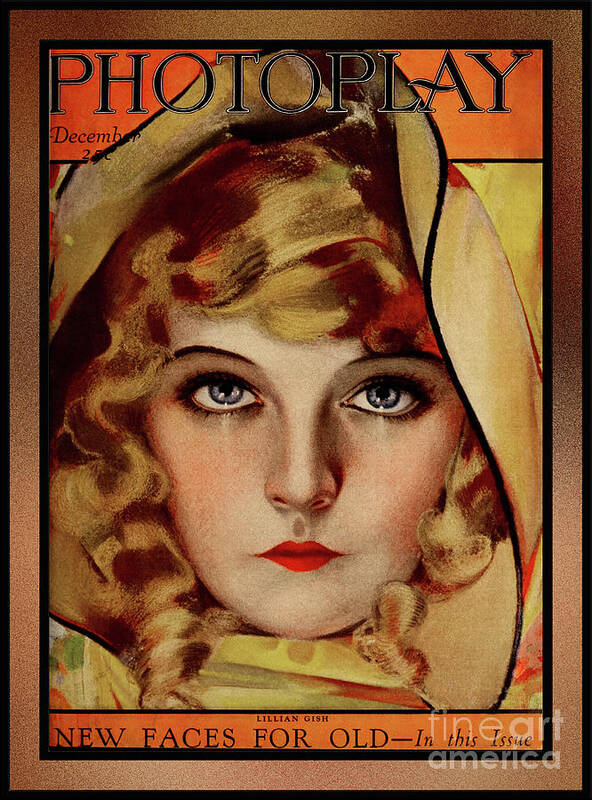The image you are seeing is a rectangular magazine cover measuring approximately six inches high by three inches wide. The cover features several borders: a thin black outer border, followed by a slightly wider bronze border that is darker in the upper left and right corners, and then another thin black border inside. 

At the top center of the magazine cover, within a red background area, is the title "Photo Play" written in black letters surrounded by white borders. Below this, on the left-hand side, the issue date "December 2nd" is printed, although some details are unclear. 

Centered on the cover, you see the face of a Caucasian woman identified as Lillian Gish, with blue-gray eyes, thin eyebrows, small red lips, and curly blonde hair. She is wearing a brown hood that covers her head, creating a somewhat solemn appearance. Her gaze is direct, looking straight into the camera.

At the bottom of the cover, there is a one-half-inch orange footer with the text "New Faces for Old – In This Issue" written in black. Over the entire cover, faintly visible, is a transparent gray watermark that reads "Fine Art America." The cover design includes a combination of beige, red, orange, yellow, brown, tan, and green colors, set against a bronze border that appears sparkly.

This cover, styled in a photo-realistic manner reminiscent of a painting, emanates a 1920s to 1930s vintage aesthetic and belongs to the publication "Photo Play," indicating an intriguing blend of visual art and magazine media.